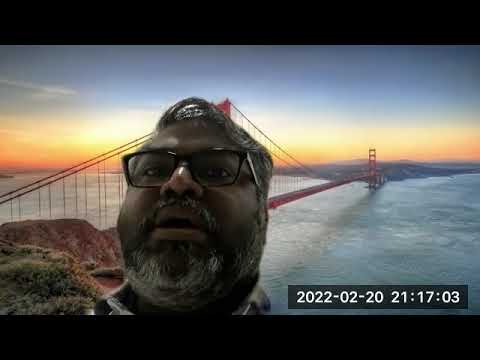The image is a vibrant, clear depiction of sunset at the Golden Gate Bridge. Framed by a sky transitioning from orange and yellow to deep blue at the horizon, the iconic bridge stretches elegantly over the water, with rocks and grass visible on the near side. In the foreground, slightly to the left of the center, the head of a dark-complexioned man with dark hair, streaked with some gray, dominates the scene. His square-rimmed, black prescription glasses frame his face which features a mustache and a beard flecked with white hairs. His head is tilted slightly backward. On the lower right corner, there's a time-stamped box that reads "2022-02-20 21:17:03." The image is bordered by a thin black strip at the top and bottom.